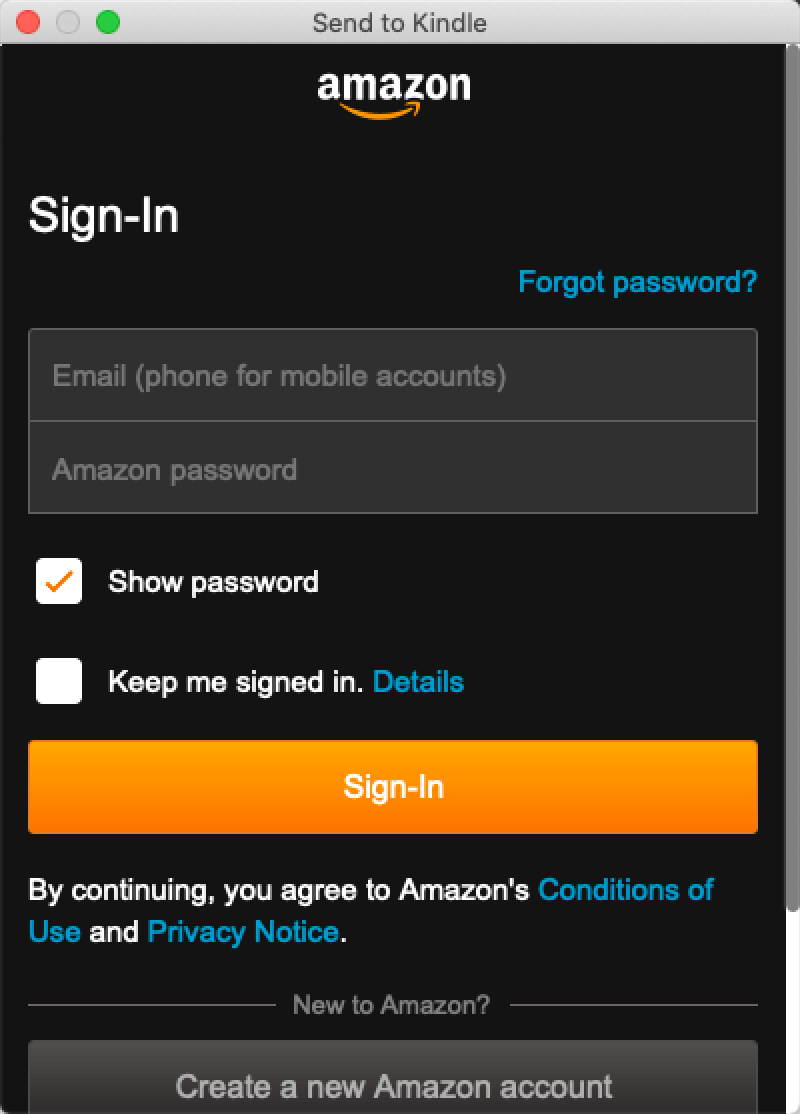A screenshot of an Amazon login page captured on a device with a black background. At the top of the screenshot, the Amazon logo is prominently displayed, followed by the heading "Sign-In." Below this, there are options labeled "Forgot Password" and "Email or mobile phone number," the latter of which is an input field for user credentials, currently shown as an empty grey block. 

Next, there is a similarly empty input field labeled "Amazon Password." Adjacent to the password field is a checkbox labeled "Show password," which allows users to see the password as they type it in. Below these fields is another checkbox with the option "Keep me signed in," accompanied by a blue link for more details.

Further down, an orange "Sign-In" button is prominently displayed. Beneath this button, there's a statement: "By continuing, you agree to Amazon's Conditions of Use and Privacy Notice."

At the bottom of the screenshot, there is a section for new customers with the prompt "New to Amazon?" followed by an invitation to "Create your Amazon account," highlighted in a way that catches the eye.